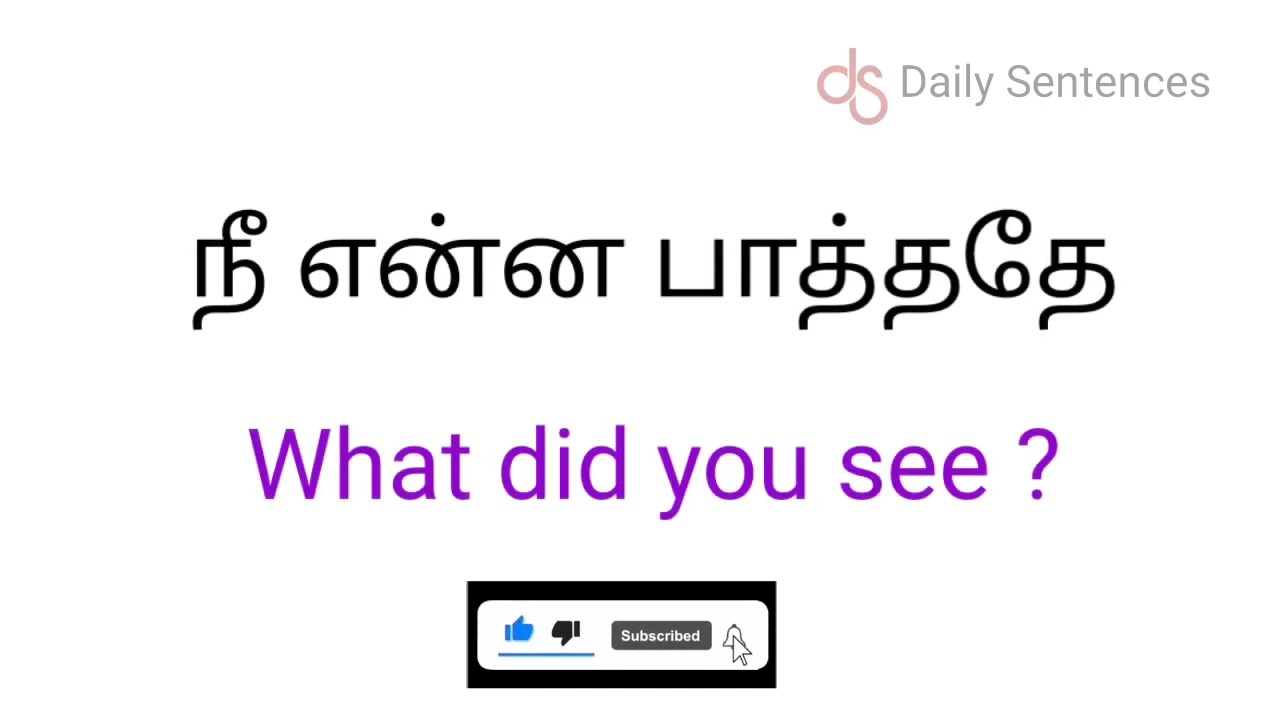This digital promotional piece is presented on a white background, devoid of any borders. The focal point at the top is the company logo featuring a stylized pink lowercase 'd' and an uppercase 'S', followed by the words "daily sentences" in gray, though slightly faded. Below this logo is a black line of text in a script resembling Arabic or another unfamiliar language, containing intricate characters including what appear to be an 'L', 'T', possible 'J's, and a formation somewhat resembling '6T'. Directly beneath this script, the question "What did you see?" is prominently displayed in purple font. At the bottom of the image is a black rectangular section featuring interactive YouTube-like icons, including a blue thumbs up, a black thumbs down, a "Subscribed" button, and a bell symbol for notifications.